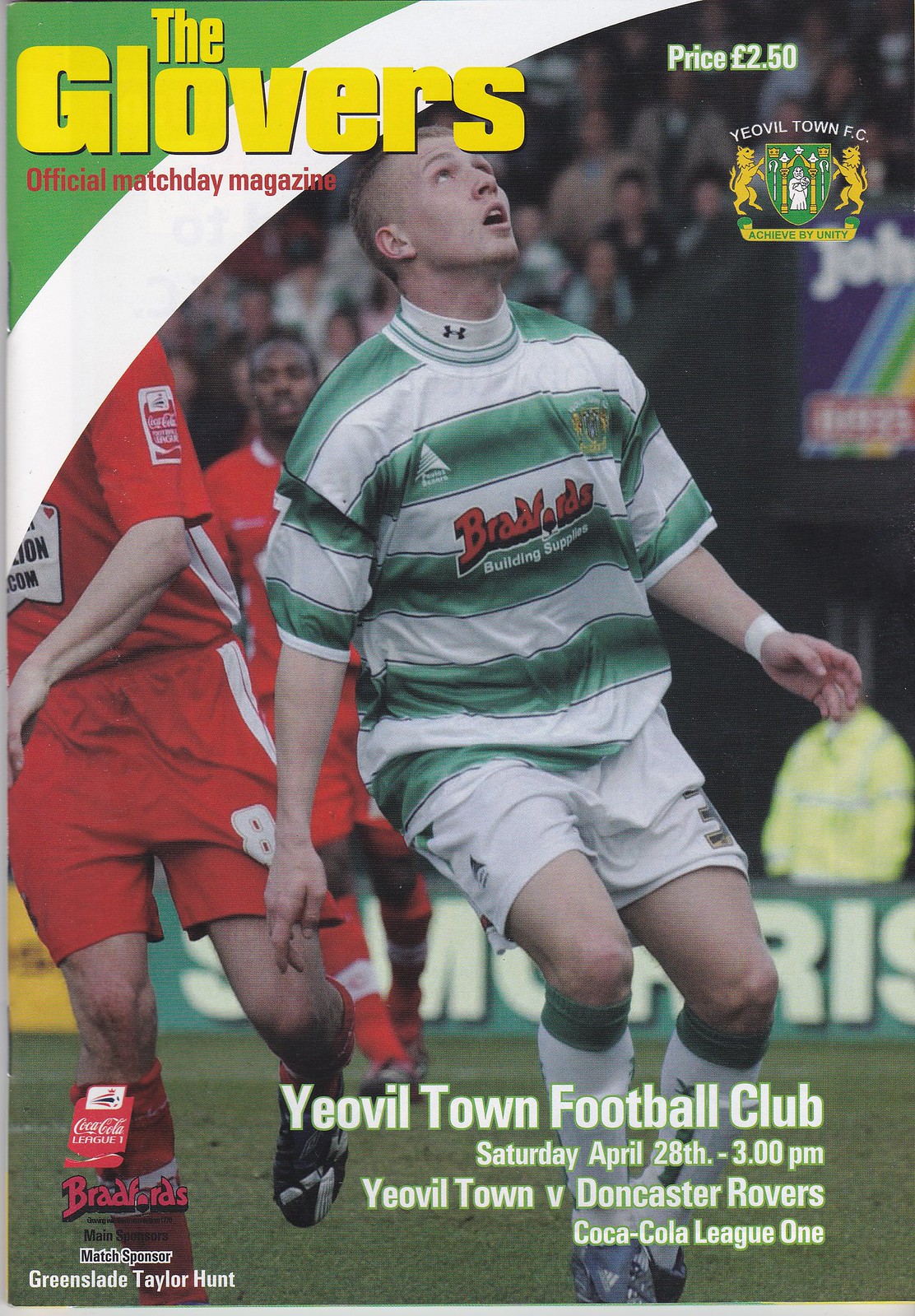The cover of the magazine features a dynamic image of a soccer match, capturing two players in action at the center. The player on the left wears a green and white striped jersey with white shorts, while the player beside him is dressed in red. Both athletes are positioned on a grassy field, with enthusiastic spectators visible in the background. At the top left corner of the cover, bold yellow text reads "The Glovers," followed by red text underneath stating "Official Match Day Magazine." Green and white ribbon-like banners add to the stylish design at the top. The top right corner displays the price, €2.50, and directly below it, the Yeovil Town FC crest is prominently featured. Additional text at the bottom of the cover announces the event: "Yeovil Town Football Club, Saturday, April 28th, 3 p.m. Yeovil Town vs. Doncaster Rovers, Coca-Cola League One." The bottom left of the cover includes sponsor logos. The entire cover showcases a vivid mix of colors, including green, yellow, red, white, black, tan, off-blue, and purple, giving it a vibrant and lively appearance.